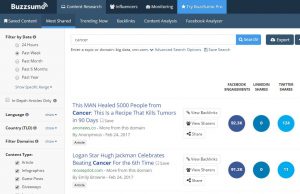The image displays a webpage from BuzzSum (spelled B-U-Z-Z-S-U-M). The page is heavily blurred (approximately 99.9% obscured). At the top of the page, there is a navy blue header featuring white hyperlinks. The lower 85% of the page has a white background with black and blue text. Positioned in the middle of the page is a search box. The visible search result includes an article titled "This Man Healed 5,000 People from Cancer." Due to the blurriness, other text on the page is not legible. On the left side, there are filtering options for search results, with discernible categories including "language" and "content type."